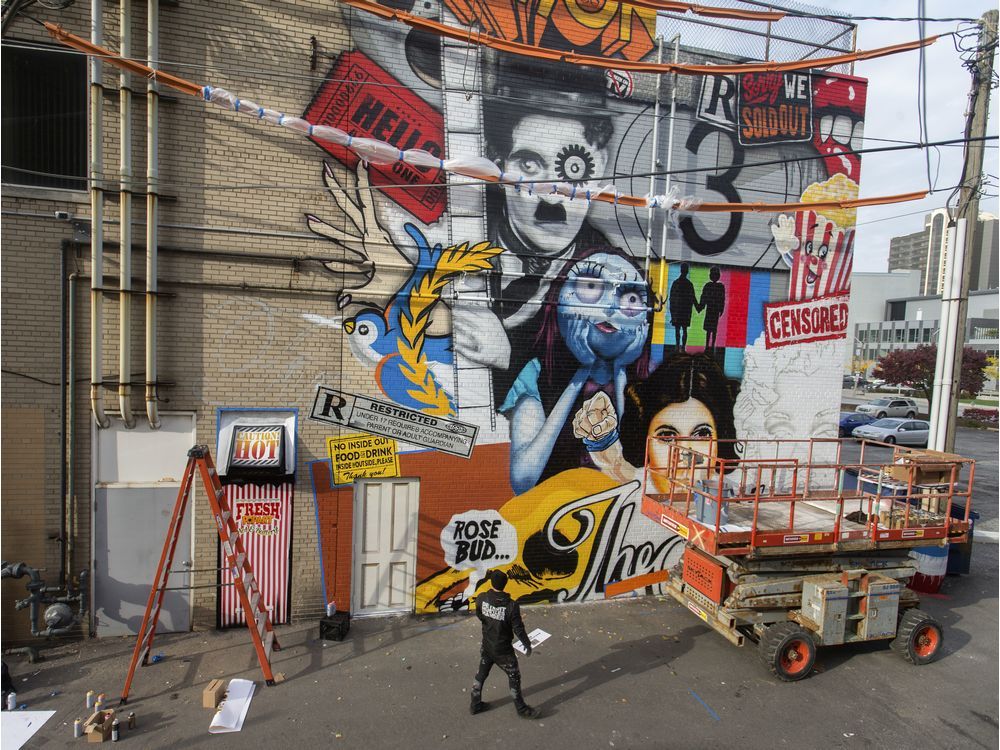The photograph captures a vibrant scene from a few stories up, showing the side of a tan brick building adorned with a colorful, spray-painted mural. The mural features an eclectic mix of movie-related imagery including Charlie Chaplin holding a film strip, a graphic illustration of a waving popcorn container with a "censored" label, a "Sorry, we're sold out" sign, a movie ticket stub, Sally from Nightmare Before Christmas, Leia from Star Wars, and a classic 3-2-1 black and white film countdown. The scene also includes a partially completed section of the mural and depicts a man on the ground wearing black pants, shoes, and a black jacket with white writing, who appears to be working on the mural. He is standing behind a scissor lift, which is red and gray with rust spots, black tires, and red wheels. The ground below him is laden with spray paint cans, and his shadow stretches across the pavement. To the left, a ladder leans against the building near some white pipes running above a silver door. The sky is crisscrossed with telephone and power lines, adding to the urban aesthetic. In the background, buildings and vehicles in softer focus suggest this is a snapshot of a smaller city corner rather than a bustling metropolis.